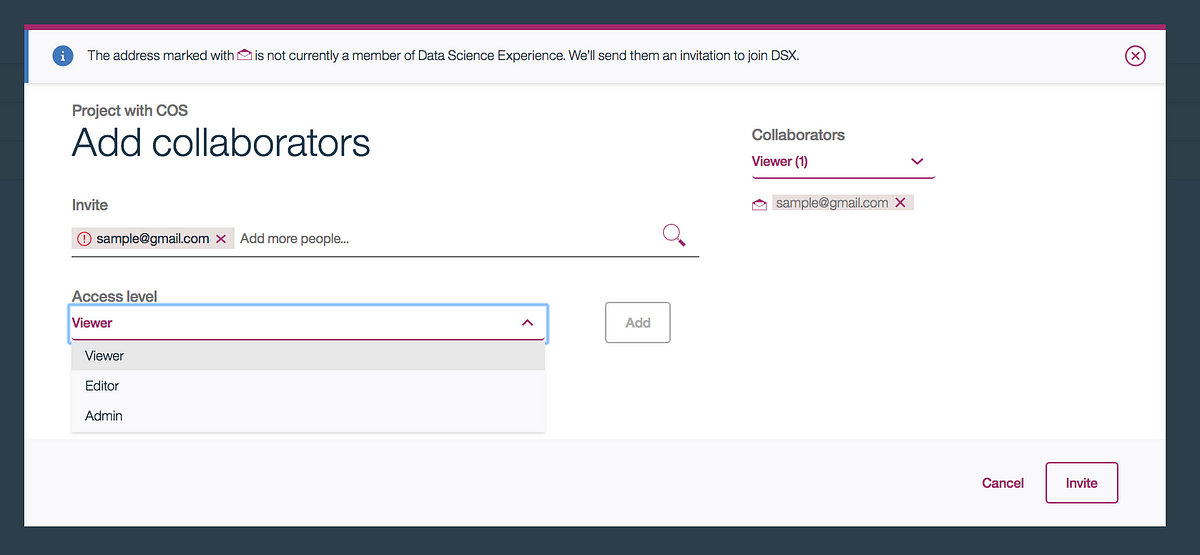The image features a user interface on a solid blue background, devoid of any additional elements. The focal point is a white window containing text and icons. A purple line accents the top of this window, while a blue line appears to the left. 

In the top section, a blue info icon generates a message stating: "The address marked with the male icon is not currently a member of the data science experience. We'll send an invitation to join GSX." This text is predominantly in black, with key terms highlighted in purple.

Below this message is the input area for adding email addresses. Currently, it displays "sample@gmail.com" and an adjacent prompt to "Add more people" to the list of collaborators. There’s also an access level dropdown menu set to "viewer," with options for "editor" and "admin" available. An "Add" button is aligned next to the dropdown menu.

To the right side, there's a section listing current collaborators. It shows "Collaborators: Viewer (1)" followed by the email "sample@gmail.com." This part organizes collaborators by their access levels.

In the bottom right corner, two interactive elements are visible: "Cancel" written in purple, and the word "Invite" enclosed within a purple box, indicating a button to send the invitation.